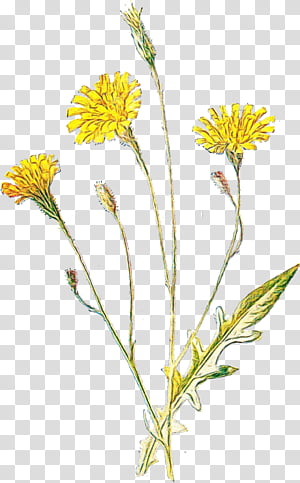The digital color illustration showcases a vertical arrangement of wildflowers set against a small gray and white checkered background. Dominating the image are three vibrant yellow flowers on long, thin green stems, each adorned with several layers of squarish petals akin to dandelions. The tallest stem features a closed bud at the very top, situated at the edge of the composition. Additional elements include three smaller buds interspersed among the primary flowers. At the base, a single, large, serrated dandelion leaf extends diagonally to the right, displaying a combination of green and yellow hues with areas appearing slightly translucent or reflective. The portrait-oriented image is meticulously hand-drawn, characterized by its clarity and bright, uplifting aesthetic, yet it remains unsigned.